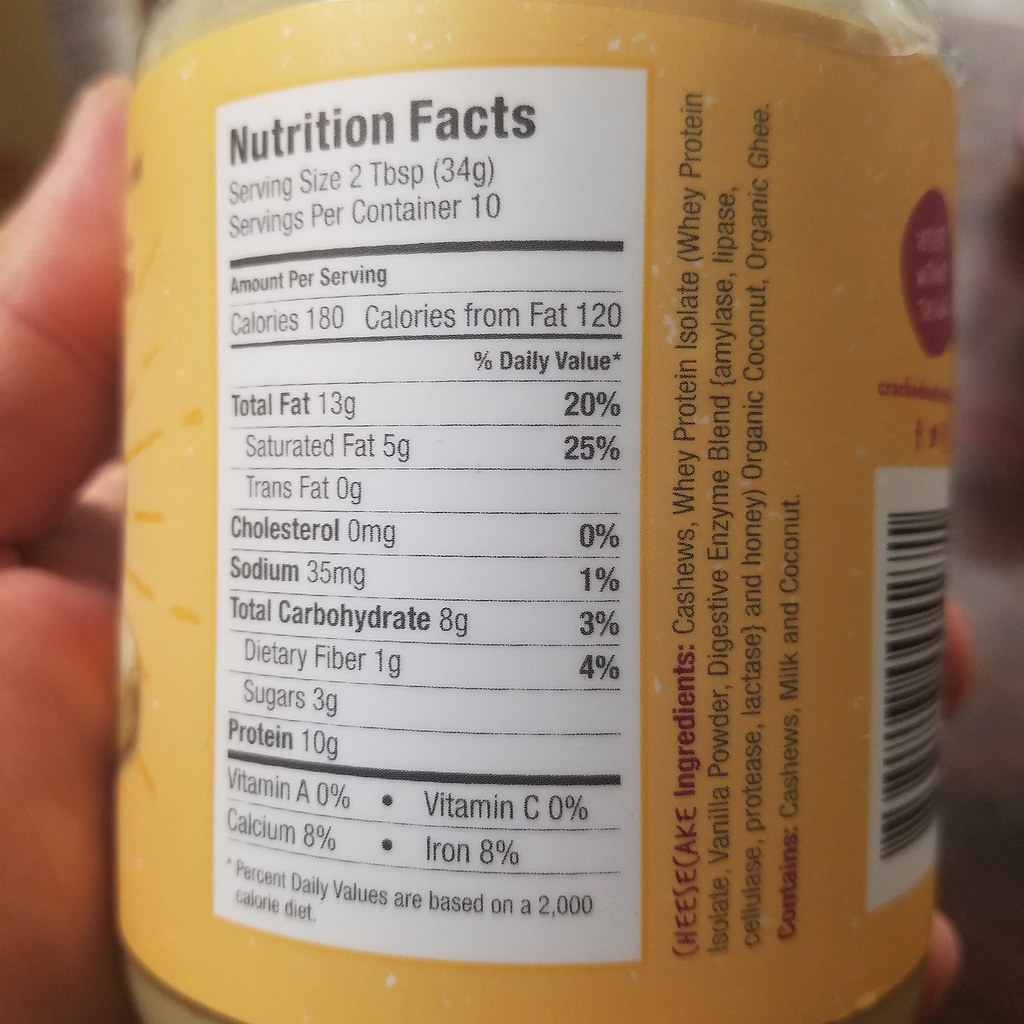In the image, a person holds a yellow-packaged bottle prominently displaying its detailed nutritional facts and ingredients labels. The nutritional facts label, printed in black lettering on a white background, showcases a serving size of two tablespoons (34 grams) and indicates that there are 10 servings per container. Key nutritional information includes 180 calories per serving, 120 of which are from fat. The label further breaks down the nutritional content by listing total fat at 13 grams (20% of the daily value), along with saturated fat, trans fat, cholesterol, sodium, and carbohydrates. It also provides percentages of the daily value for various nutrients, dietary fibers, sugars, protein (10 grams), vitamin A, calcium, vitamin C, and iron.

To the right of this label, a white-background barcode with black lines is visible. Next to the barcode, the ingredients list is clearly printed in black, specifying cashews, whey protein isolate, vanilla powder, a digestive enzyme blend, honey, organic coconut, and organic ghee (clarified butter). The label also states that the product contains cashews, milk, and coconut. Although the precise nature of the product is obscured, contextual clues like a protein content of 10 grams and a hint of a peanut illustration suggest that it could be a protein peanut butter or a similar product enriched with nuts and whey protein.